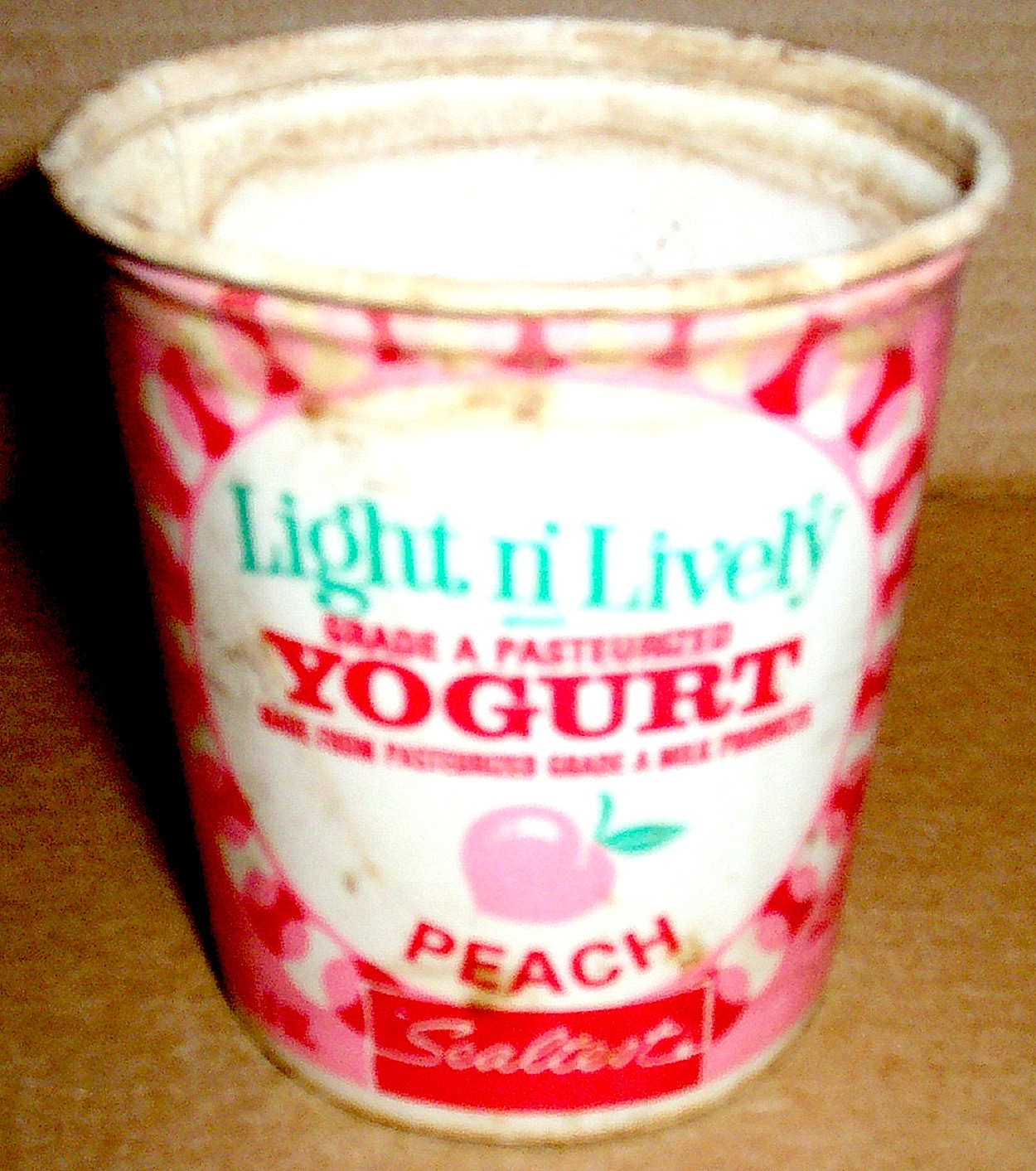In this grainy photograph, we see an old, open container of "Light and Lively" yogurt, set on a brown table or counter. The vintage container, which appears to be quite old, features distinctive design elements that haven't been used in years. Prominently displayed against a white background is the brand name "Light and Lively" in mint green text. Below this, in red lettering, it reads, "Grade A Pasteurized Yogurt, Peach Flavor." At the center of the container, there's an illustration of a peach with a small green leaf. Although the image is blurry, the words "Grade A Milk Product" seem to be discernible. Near the bottom, a red background features the word "Sealtest" in white cursive letters. The container itself, now devoid of its lid, is worn and dirty, with moldy, filthy edges and a brown-stained bottom. Adding to its vintage charm, the container is decorated with pink polka dots set against the red background.